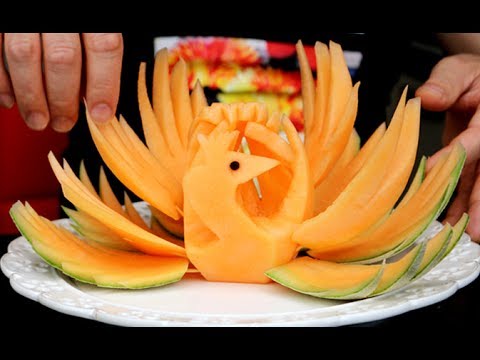The image showcases an intricately carved cantaloupe displayed on a white plate, framed by black borders at the top and bottom. The cantaloupe, with its delicate carvings, features a central figure that morphs from what appears to be a snake or possibly a bird, extending out to the sides like intricate feathers or tendrils. Each section of the cantaloupe is meticulously carved, with stalks protruding from the center. The cantaloupe itself is orange with a green outer edge. 

Foregrounding this culinary artwork, two hands are visible, gently grasping the plate—three fingers on the left and a thumb with part of two fingers on the right. In the background, a person stands, partially visible, adorned in a black jacket and a multicolored shirt. This detailed craftsmanship not only highlights the talent involved but also the patience and precision required to create such a beautiful sculptural piece.